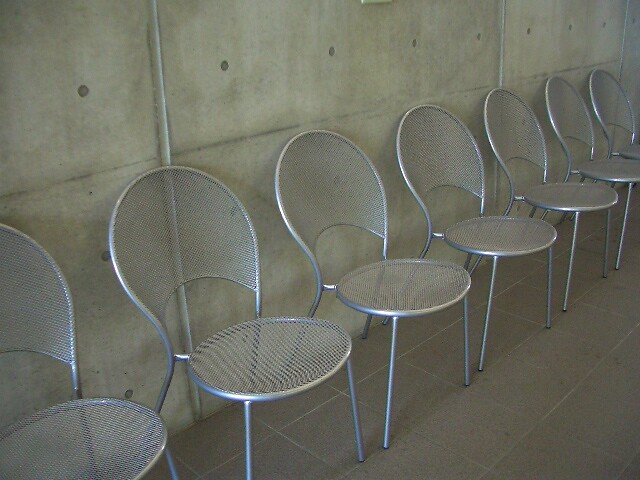In this photograph, we see seven identical aluminum-framed chairs arranged in a single, evenly spaced row. Each chair is positioned flush against a heavy concrete wall adorned with small gray circles. The wall features vertical silver-colored metal support bars that may be part of its structure. The chairs, all seemingly brand new without any scratches or blemishes, are distinguished by their metal mesh round backrests with gaps between the seat and back, and round seats without cushions or armrests. The floor beneath them is tiled in a medium to dark gray shade, showing no signs of major wear or damage, only minor imperfections. The overall setting suggests an industrial or warehouse environment rather than a domestic one.